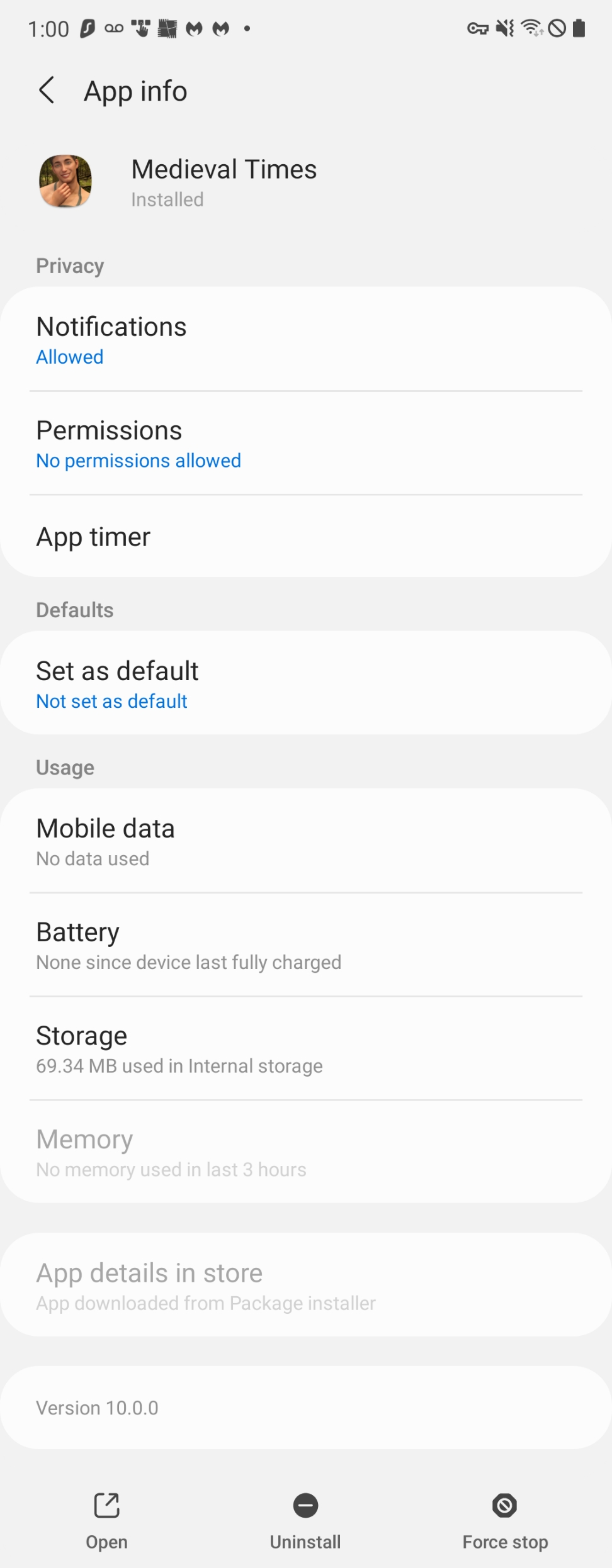The image appears to be a screenshot of a smartphone displaying detailed information about an installed app named "Medieval Times." The time shown at the top of the screen is 1 o'clock. There are several icons visible, including ones for Malwarebytes and voice messages. The section below displays the app's details, including a thumbnail image of a smiling man with light brown skin and possibly dark hair, which is likely an icon representing a character in the game. 

The screen reads, "App Info" followed by multiple informational headings:
- "Privacy"
- "Notifications," marked with "Allowed" in blue
- "Permissions," showing "No permissions allowed" in blue text
- "App Timer" and "Defaults," with "Set as default" in black and "Not set as default" in blue
- "Usage," indicating "Mobile data" in black and "No data used" in gray
- "Battery," noting "Nonsense device last fully charged" in gray text
- "Storage," specifying "69.34 MB used in internal storage" in gray text
- "Memory," with "No memory used in last three hours" in gray text
- "App details in store" states the app was downloaded from the package installer, with a version number of 10.0.0

At the bottom, the screen provides three actionable buttons arranged horizontally:
- "Open"
- "Uninstall"
- "Force Stop"

This screenshot offers a comprehensive view of the game settings for "Medieval Times" as seen on the user's phone.